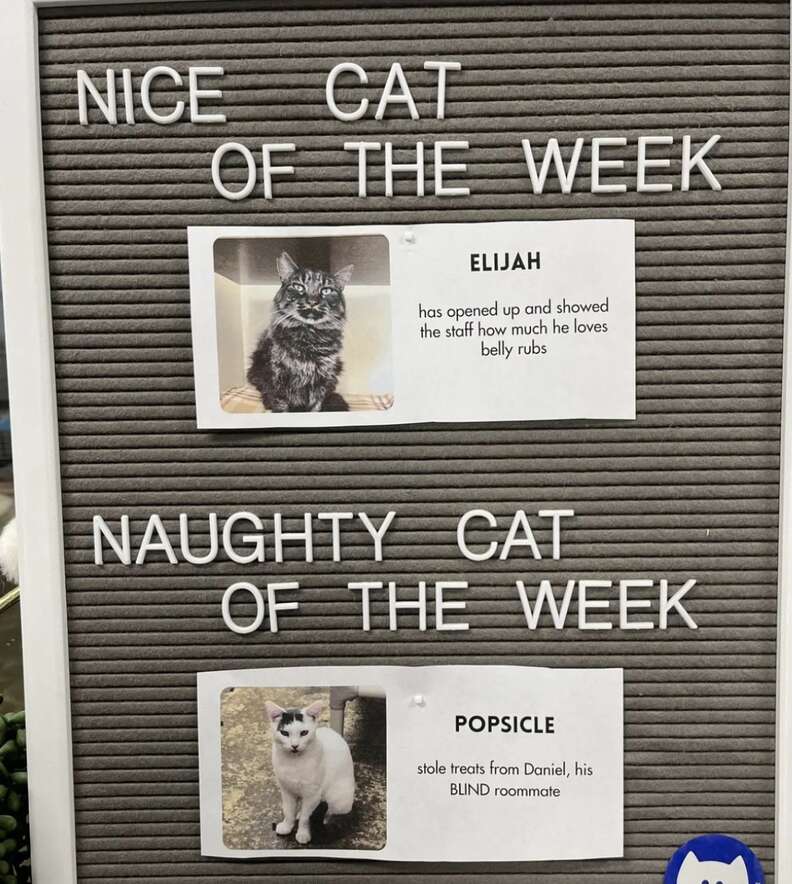The image depicts a menu board-like display in what seems to be an animal shelter or pet care facility. The board has a dark gray or blackish background with a white frame. At the top, white plastic letters spell out "Nice Cat of the Week". Below this heading is a picture of a gray and white cat with blue eyes named Elijah. Next to Elijah's picture, text reveals that Elijah has "opened up and showed the staff how much he loves belly rubs."

Further down on the board, also in white letters, is the heading "Naughty Cat of the Week". Beneath this, a white triangular piece of paper displays a picture of a white cat with a small black patch on his head. This cat is named Popsicle, and the text states that Popsicle "stole treats from Daniel, his blind roommate." There is also a blue circular insert at the bottom right corner of the board. The entire setup allows for the text to be changed easily and serves as a playful feature within the pet care environment.